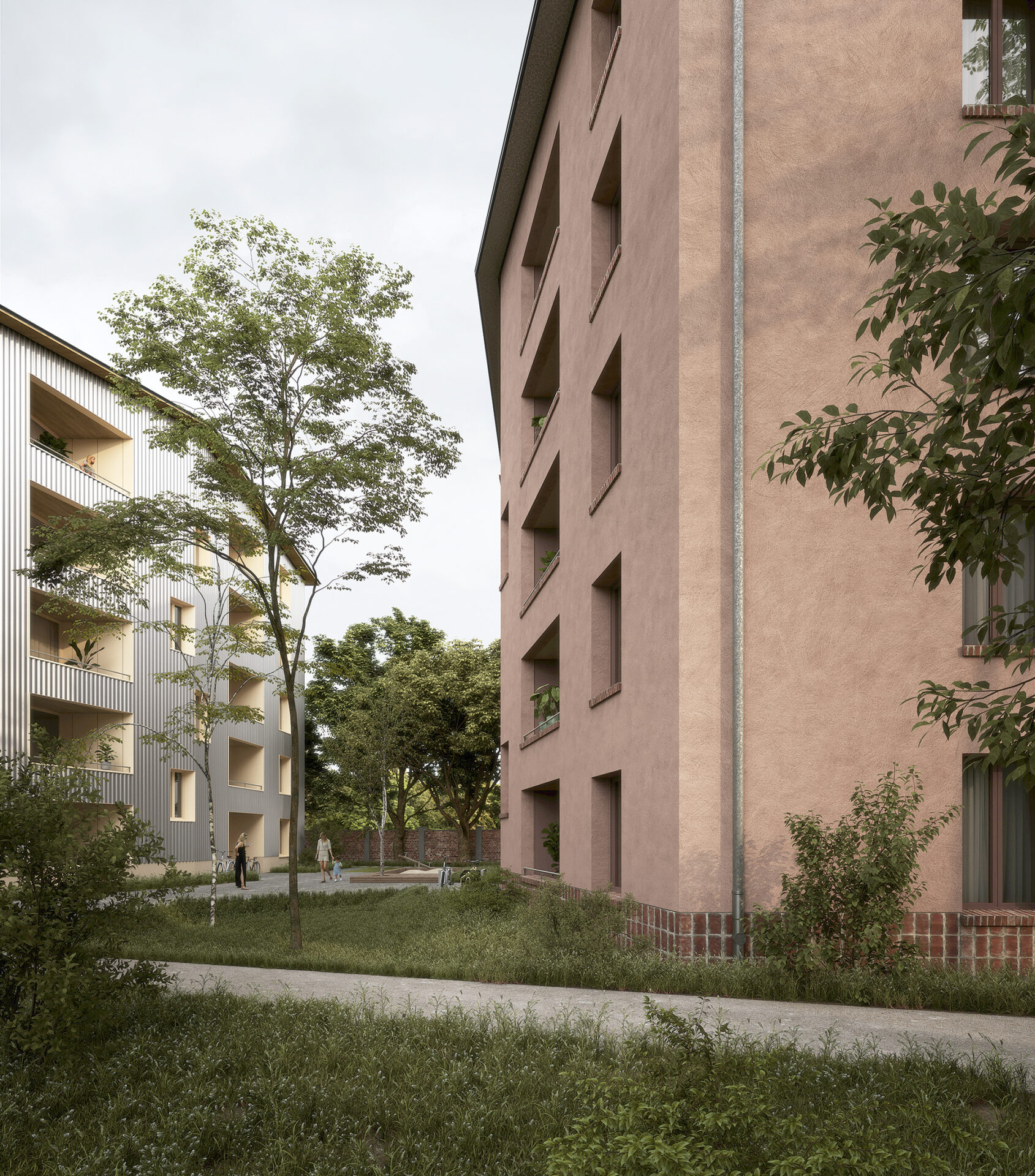This outdoor photograph showcases a complex with two tall, multi-story buildings facing each other across a landscaped plaza. The building on the right is prominently beige with reddish-brown brick lining its base. Its smooth exterior features several rectangular openings serving as balconies, accented by a vertical gray pipe running up its side. Adjacent to it on the left is a white building with many balconies and verandas, featuring beige walls. Notably, the top veranda on the left side of this building has a person peering out, adding a touch of life to the scene.

The plaza itself is vibrant with greenery, including a tall tree that, from the photograph's perspective, appears taller than the buildings, though it isn’t. Below this tree is a bush, and a variety of plants and grass cover the front section of the image. There is also a smaller tree situated between the buildings, and off to the right side, another tree just comes into view. 

In the foreground, a woman with blonde hair in a black dress is seen holding the hand of a small child who stands beside a sandbox lined with brown bricks. Beside them, a concrete sidewalk winds through the plaza, cutting off at the bottom of the image and reappearing near where they are standing. The sky overhead is gray and overcast, but the scene remains brightly lit, adding to the inviting atmosphere of this residential complex.